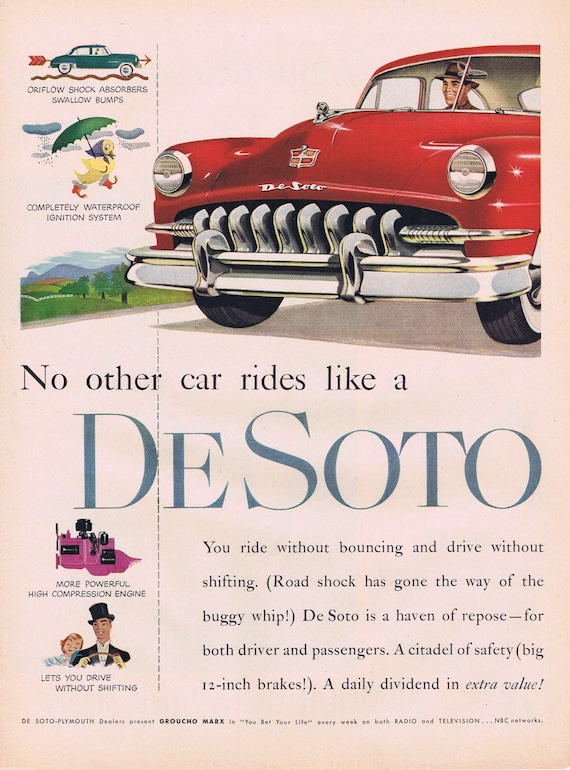This is a detailed vintage advertisement from the 1950s featuring a DeSoto automobile. The vertically oriented page appears to be from a magazine and showcases a professionally illustrated ad rather than a modern photograph. The centerpiece is a striking red DeSoto car, with a happy cartoon man driving and prominently displayed chrome front grille and headlights.

To the top left of the ad, a smaller inset features a green car with a red arrow piercing through it, accompanied by the text "OriFlow Shock Absorbers, Swallow Bumps." Below this, a whimsical yellow chick is illustrated marching in the rain with a green umbrella and a purple scarf, emphasizing the "completely waterproof ignition system."

The main text of the advertisement, written in large blue letters, declares, "No other car rides like a DeSoto." Additional promotional slogans are peppered across the ad, such as "You ride without bouncing and drive without shifting," "Road shock has gone the way of the buggy whip," and "DeSoto is a haven of repose for both driver and passengers." There’s also mention of its "more powerful high compression engine" and the innovative feature that lets you drive without shifting, which suggests the car is automatic.

The background of the ad features a scenic landscape of hills, mountains, and trees, adding to the feeling of a serene and enjoyable driving experience. The vibrant color palette includes shades of red, green, blue, yellow, pink, and silver, enhancing the liveliness of the vintage illustration. Overall, the ad evokes a sense of nostalgia and showcases the DeSoto as a symbol of comfort, innovation, and safety in mid-20th-century automobile engineering.